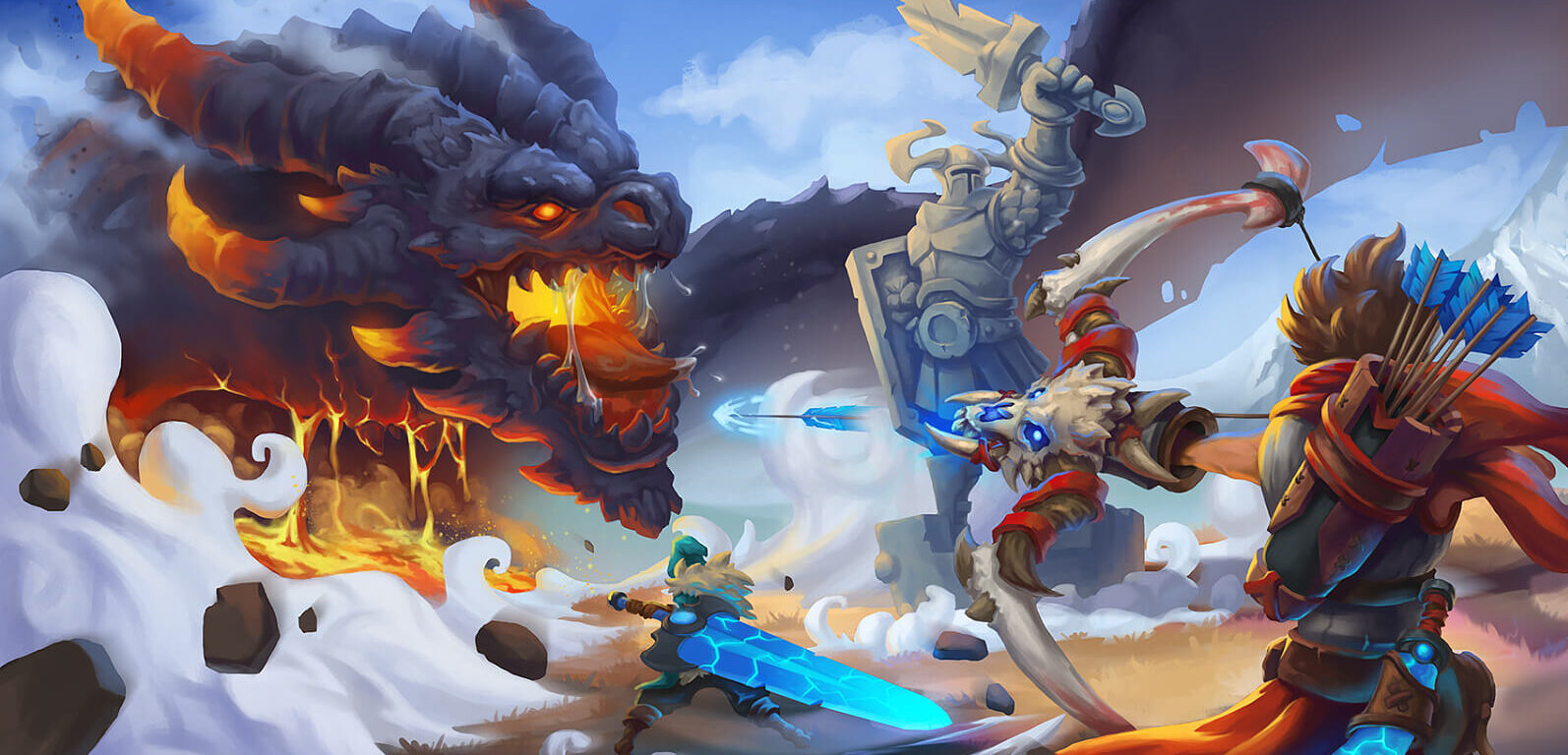The image depicts a vivid, cartoonish action scene reminiscent of a video game illustration set against a clear blue sky. Dominating the upper left corner is a colossal dragon-like creature with a fierce, charcoal-gray head adorned with horns, glowing red eyes, and numerous jagged edges. The dragon's mouth is agape, revealing flames and molten lava within, with cracks on its chin and chest spewing lava, and smoke or haze trailing beneath it. On the ground, there are white patches of snow and rocky terrain leading into distant mountains. 

In the foreground, towards the lower right corner, stands an archer in a futuristic red and blue uniform, poised to shoot an arrow from a bow decorated with a skull motif. The archer's blue quiver is visible. At the center of the scene is a silver-armored knight wielding a massive, cracked blue sword. Both characters face away from the viewer, with the knight sporting blonde hair.